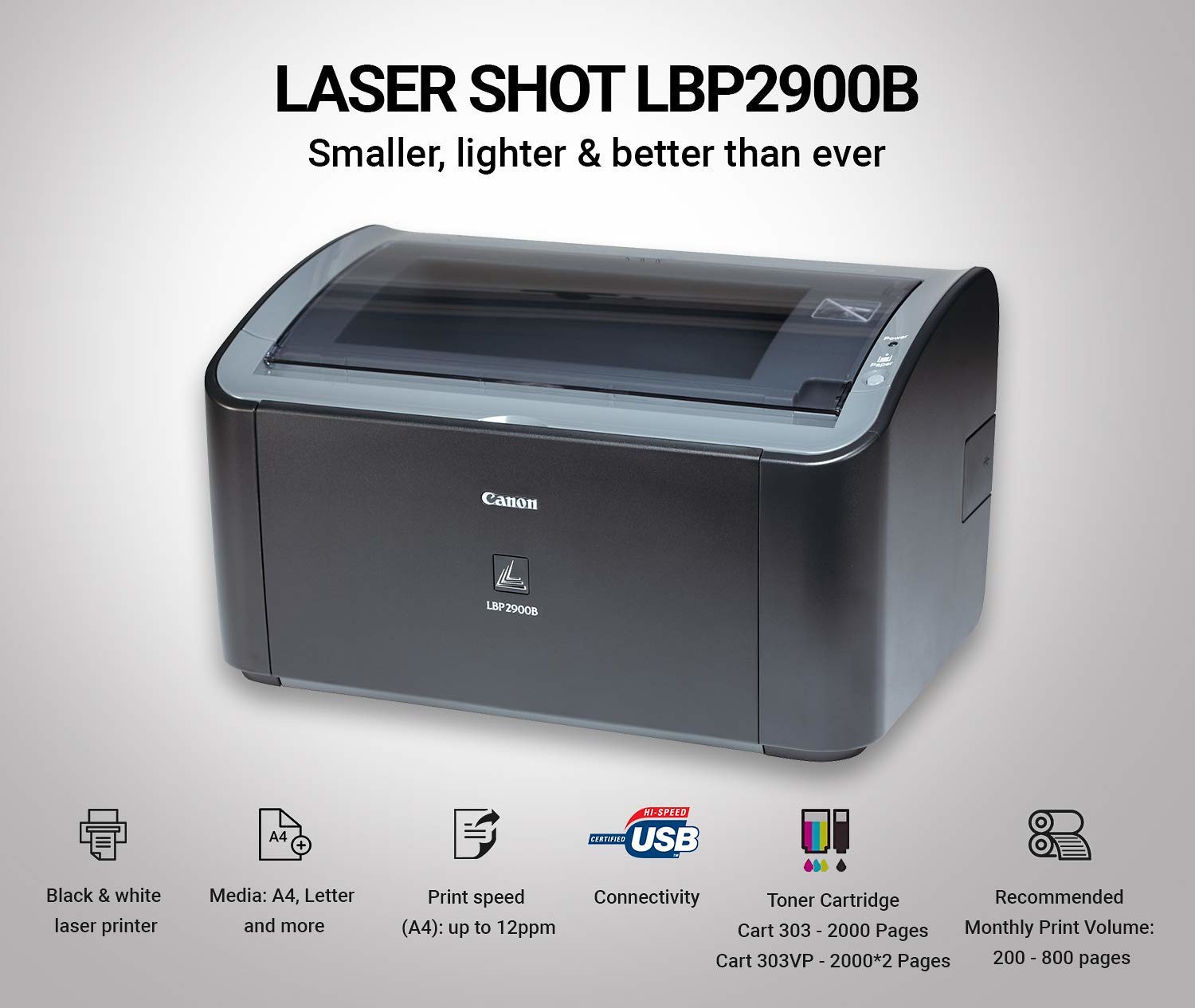The image is an advertisement for the Canon LaserShot LBP2900B printer, featuring a sleek, compact, and modern design in black and gray tones with a shadow effect. The printer image prominently occupies the center, and it's topped with the text "LaserShot LBP2900B" in bold black capitals. Beneath this, a subtitle reads "Smaller, lighter, better than ever" in smaller black text, emphasizing the printer's improvements.

The bottom left corner features several icons and text descriptions in red, white, and blue colors, highlighting the printer's key features. These include:

- A black and white laser printer logo.
- A media compatibility icon indicating A4, letter, and more paper sizes.
- An A4 print speed specification of up to 12 ppm.
- A high-speed USB connectivity icon.
- Toner cartridge details: "Cart 303 - 2,000 pages" and "Cart 303VP - 2,000 x 2 pages," accompanied by an ink symbol.
- A recommended monthly print volume range of 200-800 pages.

The advertisement's background is a plain gray, enhancing the visual focus on the printer and the accompanying information.